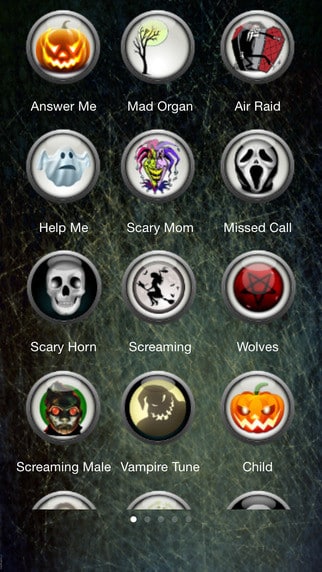The image appears to be of a digital device, possibly a cell phone or a tablet, displayed on a weathered background with a gradient from darker bluish-green at the top to a lighter bluish-green at the bottom. The surface has a distressed texture resembling scratches. The device's screen showcases several rows of circular icons, each with a shiny appearance and a gray metallic outline.

At the top of the screen, partially cut off, are several rows of icons:
- The first visible icon is labeled "Answer Me."
- Below it, icons are labeled "Mad Organ" and "Air Raid."
- The next row includes "Help Me," "Scary Mom," and "Miss Call."
- Further down are icons titled "Scary Horn," "Screaming Wolves," "Screaming," "Male Vampire," "Tune," and "Child."

The icons have a variety of colors, including orange, black, green, yellow, red, purple, pink, white, gray, and multiple shades of red and green. Given the assortment of labels and vibrant colors, these icons likely represent various apps or games.